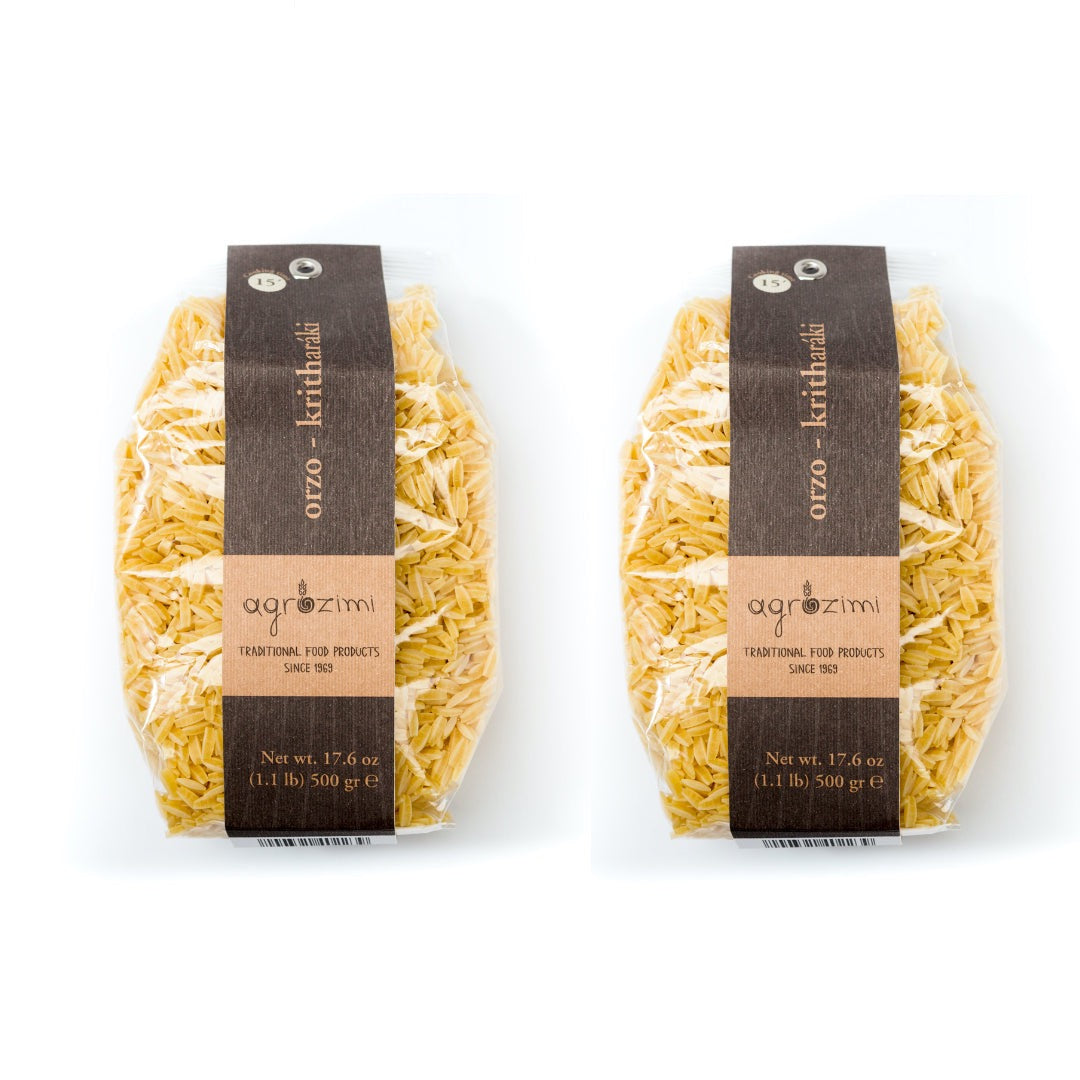The image is a color photograph displaying two identical packages of orzo pasta set against a solid white background. Each package is made of clear plastic, revealing the small, rice-shaped pasta inside, which is a golden-yellow color. The packages feature a vertical band label that runs down the middle. The label is predominantly dark brown with a square section of reddish-brown in the center. The label includes the product name "Agrosimi" in a stylized font, and below that, "Traditional Food Products Since 1969" in a black homemade font. Towards the bottom, the label mentions the weight of the package: 17.6 ounces (1.1 pounds or 500 grams). Additionally, there is a small silver tab at the top of the label and a barcode located at the very bottom of each package.